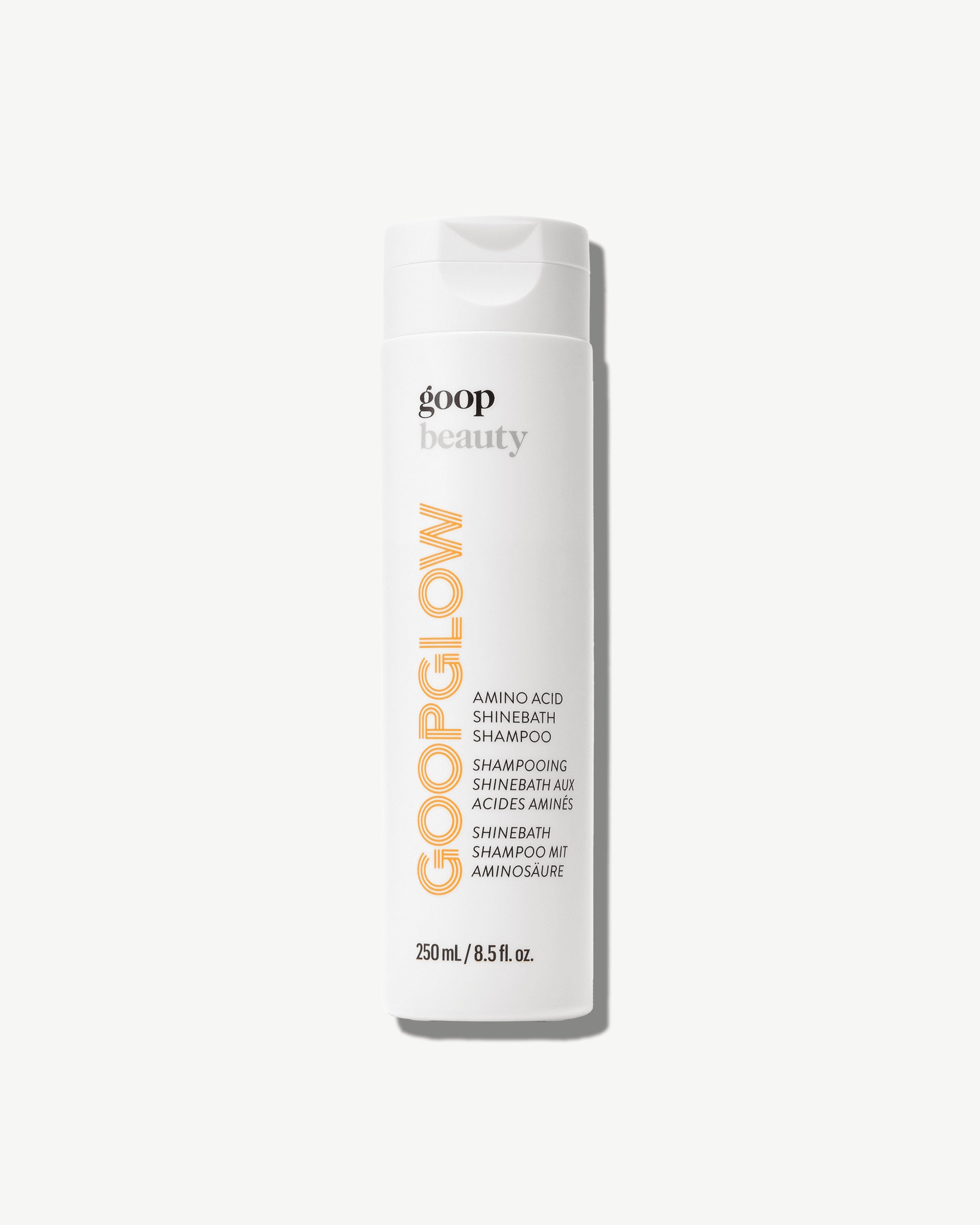This product image features a white tube of Goop Beauty's Goop Glow Amino Acid Shine Bath Shampoo, set against a solid white background. The tube displays the brand name "GOOP BEAUTY" at the top in black and gray. Running vertically in large, orange, all-capital letters is the product line name "GOOP GLOW." To the right of this, the product description "Amino Acid Shine Bath Shampoo" is printed in smaller, all-capital, black letters, accompanied by its French translation "Shampooing Shine Bath AUX ACIDES AMINÉS" and its German translation "SHINE BATH SHAMPOO MIT AMINOSÄURE." At the bottom of the tube, the volume is specified as "250 milliliters / 8.5 fluid ounces." The tube has a closed flip-off cap that casts a faint gray shadow, adding depth to the otherwise minimalist white background. There are no other texts, products, or context elements present in the image.